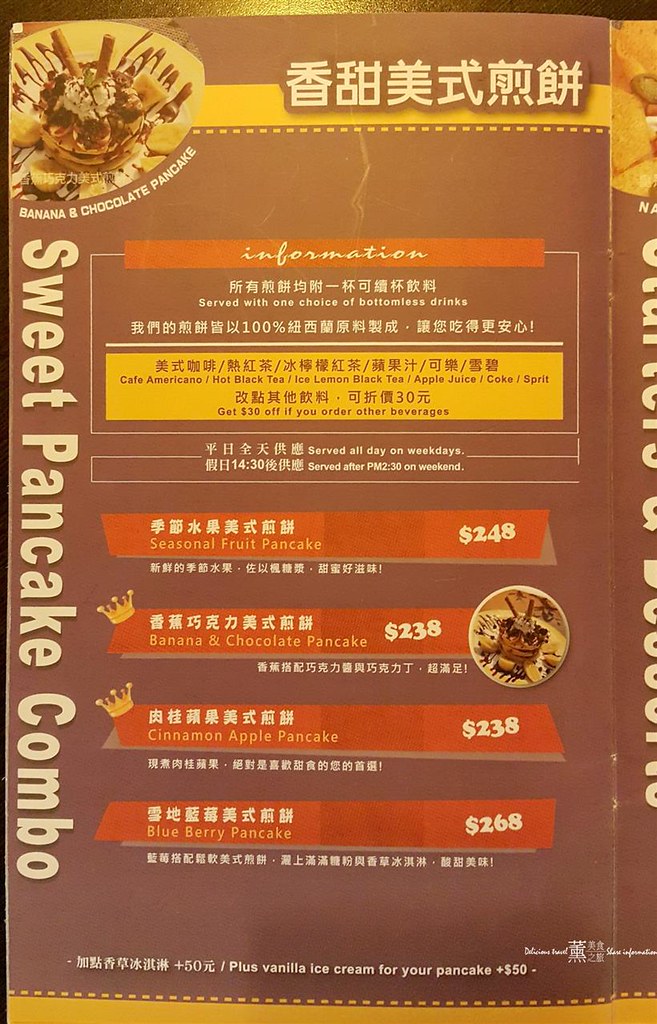This vertically-oriented color photograph captures a section of a breakfast menu, rendered with a warm, yellowish tint due to artificial tungsten lighting. The left side of this menu prominently features both English and an Asian language, possibly Korean, Chinese, or Japanese. At the top left corner, an enticing photograph displays "Banana and Chocolate Pancakes"—a decadent plate topped with generous amounts of bananas and drizzled with hot fudge. Below this image, the text "Sweet Pancake Combo" runs along the left edge. The top menu item is highlighted in a white text box, and the item headings are presented on orange banners, two of which are adorned with a crown icon on the left. Prices of menu items are clearly listed, with examples including $2.48, $2.38, and $2.68. The overall composition suggests a detailed and appealing presentation of breakfast options.